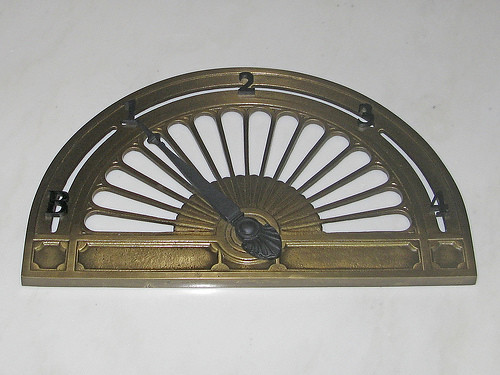The photograph captures a vintage elevator floor indicator laid out on a white surface. The brass or bronze semicircular device, resembling a fan, features a design reminiscent of peacock feathers carved into its structure. The indicator has a black pointer currently directed at the number "1." Along the outer edge of the semicircle, there are floor numbers and a letter positioned symmetrically: a "B" for basement on one end, followed by "1," "2," "3," and "4" in ascending order. The intricate design along the bottom includes various rectangles and small holes, enhancing its ornate, old-fashioned appearance.